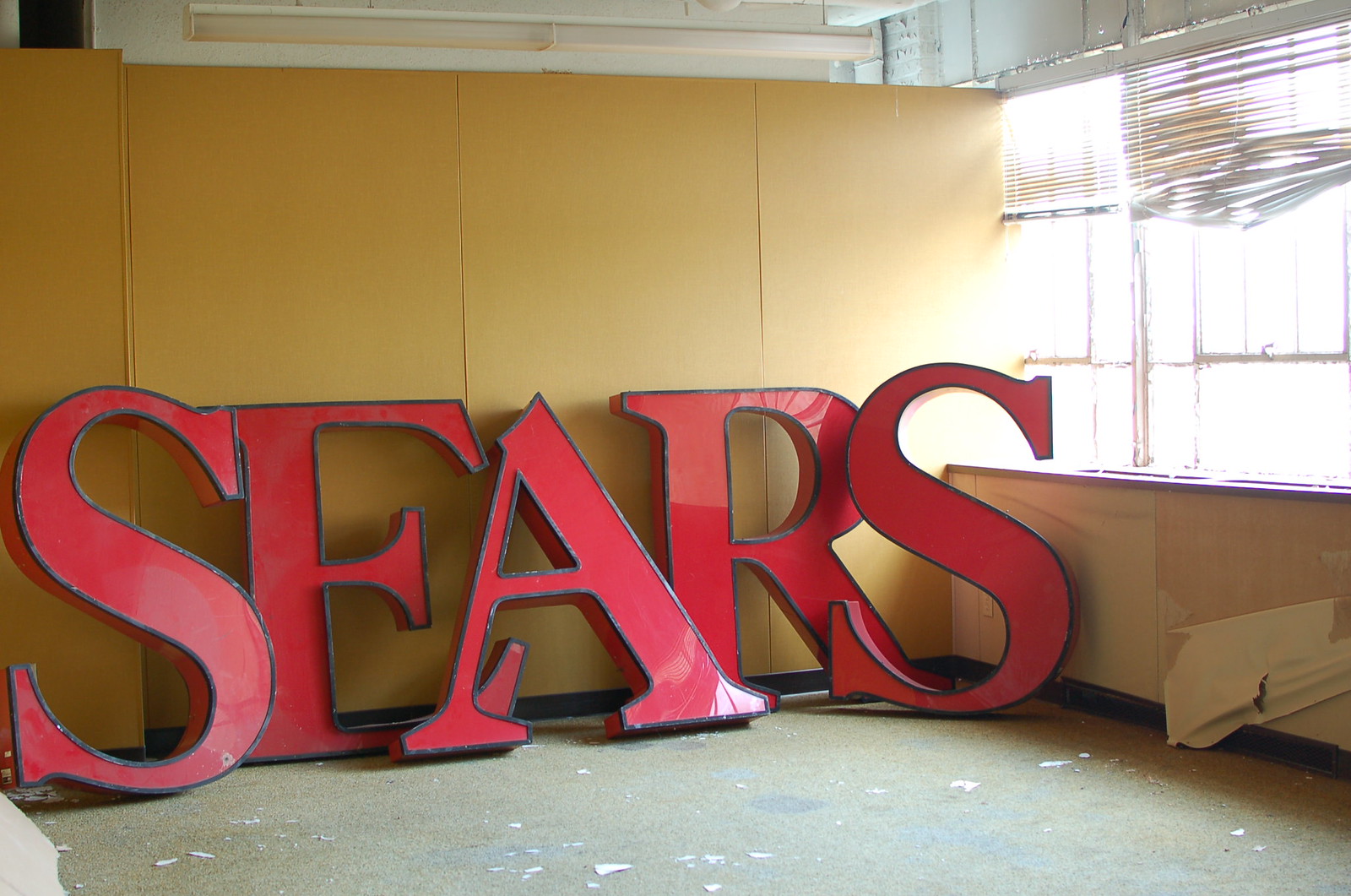The photograph captures an indoor room undergoing renovation. On the right side, a series of windows adorned with horizontal, thin blinds is visible; while most of the blinds are pulled up, the blinds on the far-right window appear damaged and hang loosely in the middle. Below the windows, a segment of beige wallpaper is noticeably peeling off the wall, exposing what appears to be an unfinished surface underneath. The room’s back wall is also covered with the same beige wallpaper. 

Positioned on the concrete floor are large, bold red letters spelling out "Sears," with each letter outlined in black. The floor itself is scattered with small scraps of paper, indicative of ongoing renovation work. The ceiling, primarily off-white, features a single visible light fixture. Overall, the scene conveys the impression of disarray and transition, highlighting the room's current state of refurbishment.